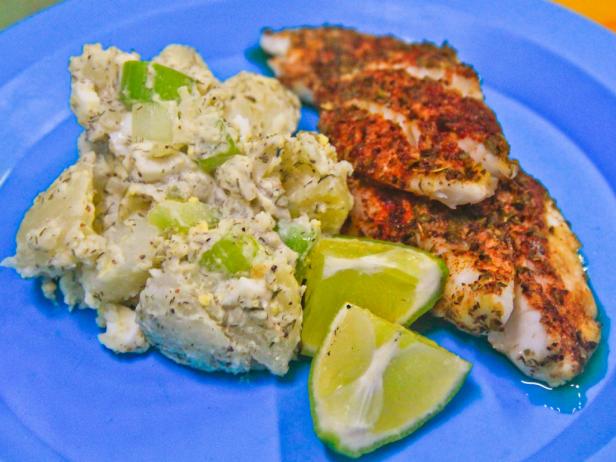This detailed photograph showcases a beautifully arranged meal on a cornflower blue plate. On the right-hand side, two golden-brown, breaded chicken breasts are cooked to perfection, hinting at a crispy exterior. Nestled between the chicken breasts and the potato salad on the left are two lime wedges, likely intended for a zesty garnish. The potato salad itself appears rich and creamy with generous amounts of mayonnaise, speckled with crunchy vegetables like green peppers, celery, and potentially onions. A subtle hint of oil can be seen seeping around the base of the chicken, adding an appetizing glisten. In the background, there are pops of tangerine and green colors on the upper right and left corners, adding a touch of vibrancy to the scene. The overall portion size of the meal is comparable to the span of two adult hands, making it a hearty serving.